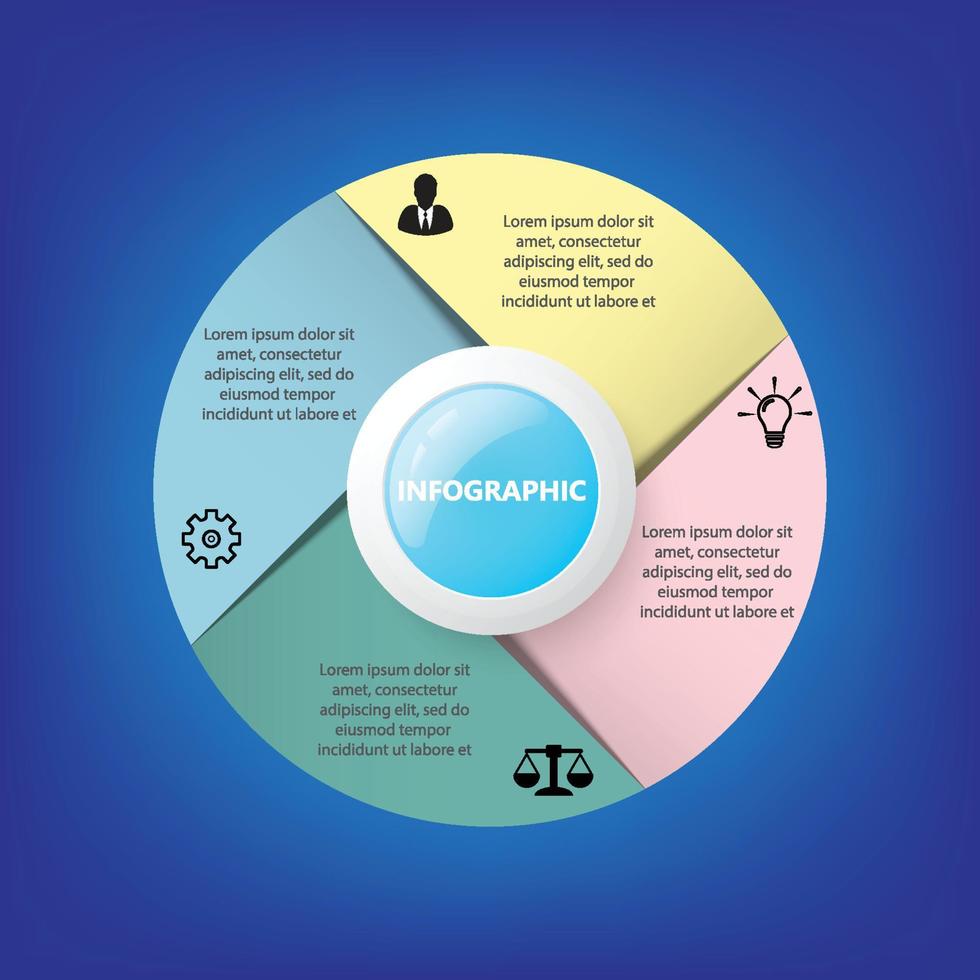This infographic features a prominent blue background with a central circular design. At the core, a smaller circle in light blue displays the word "infographic" in white text. Surrounding this inner circle, a larger white circle is segmented into four equal quadrants, each distinguished by a different color – yellow, pink, green, and blue.

Each of the four sections contains identical Latin placeholder text starting with "Lorem ipsum, dolor sit, amet,” spread across five lines. The quadrants also feature distinct icons, each set against a colored triangular backdrop:
- The top yellow section at 12 o'clock depicts a silhouette of a man wearing a suit and tie.
- The pink section at 3 o'clock showcases a lit light bulb with radiating lines.
- The green section at 6 o'clock displays a balanced scale, symbolizing justice.
- The blue section at 9 o'clock features a gear, representing settings or mechanics.

All icons are rendered in black, standing out starkly against their colored backgrounds, creating a clear, organized, and visually appealing infographic template.